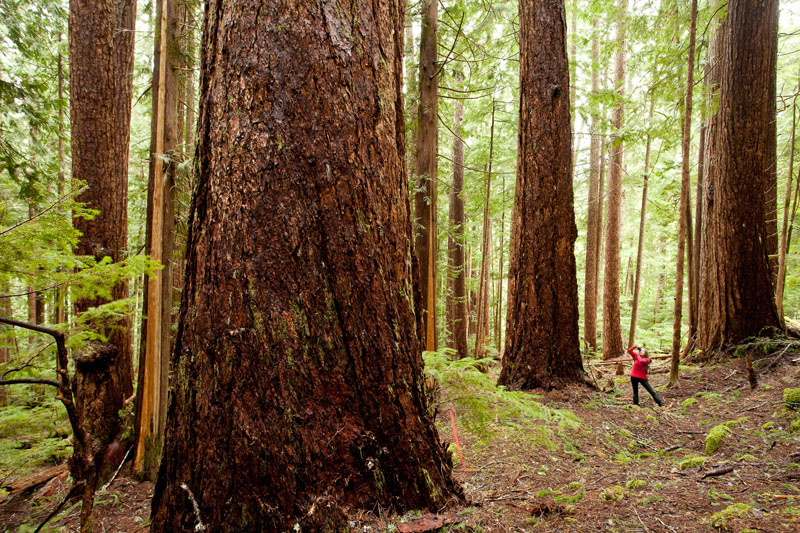The photograph captures the immense grandeur of a forest, dominated by enormous, towering tree trunks with thick, brown bark. The sheer size of these trees is awe-inspiring, dwarfing the lone person in the image, who is dressed in a red long-sleeved shirt and black pants. She stands in the background, taking a picture of the colossal trunks. The forest floor is a mixture of dirt, small branches, twigs, and green weeds, accented with patches of brown, dead grass. To the left of the image, a few leaves are visible, while smaller, thinner trees with green leaves grow up in the background, contributing to the dense forest scenery. Through the trees, slivers of sky with white light shine down, highlighting the depth and complexity of the woodland environment.